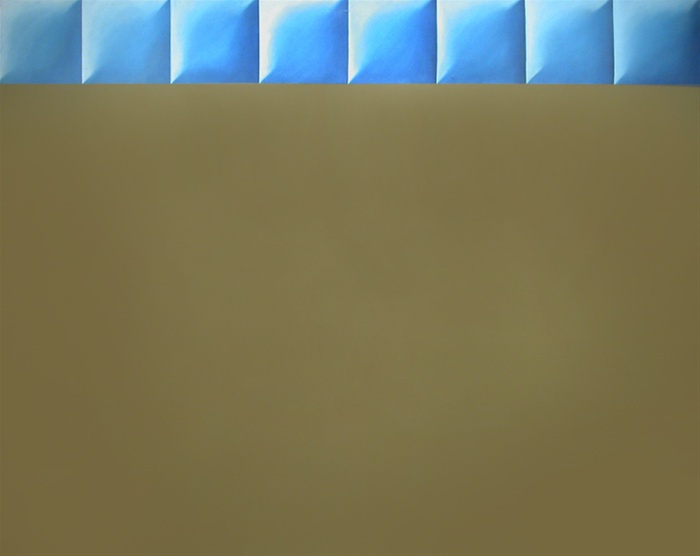The image depicts a wide rectangular scene with a predominantly dull gold or bronzy-brown background, which appears to measure approximately eight inches wide by seven inches tall. The upper portion of the image features a row of eight square tiles that resemble Tetris blocks or computer-generated 3D cubes. These tiles are primarily light blue, but the hue transitions slightly; the leftmost and rightmost tiles have a more grayish-blue tone, while the second tile from the left is a bit lighter. The third through seventh tiles exhibit a shiny white highlight on their left sides. Each tile is marked by a diagonal line stretching from the bottom left corner to the top right corner, along with a faint circular imprint. The overall image has no additional objects, text, or fonts, and features subtle shading or gradient effects on both the tiles and the brown background.